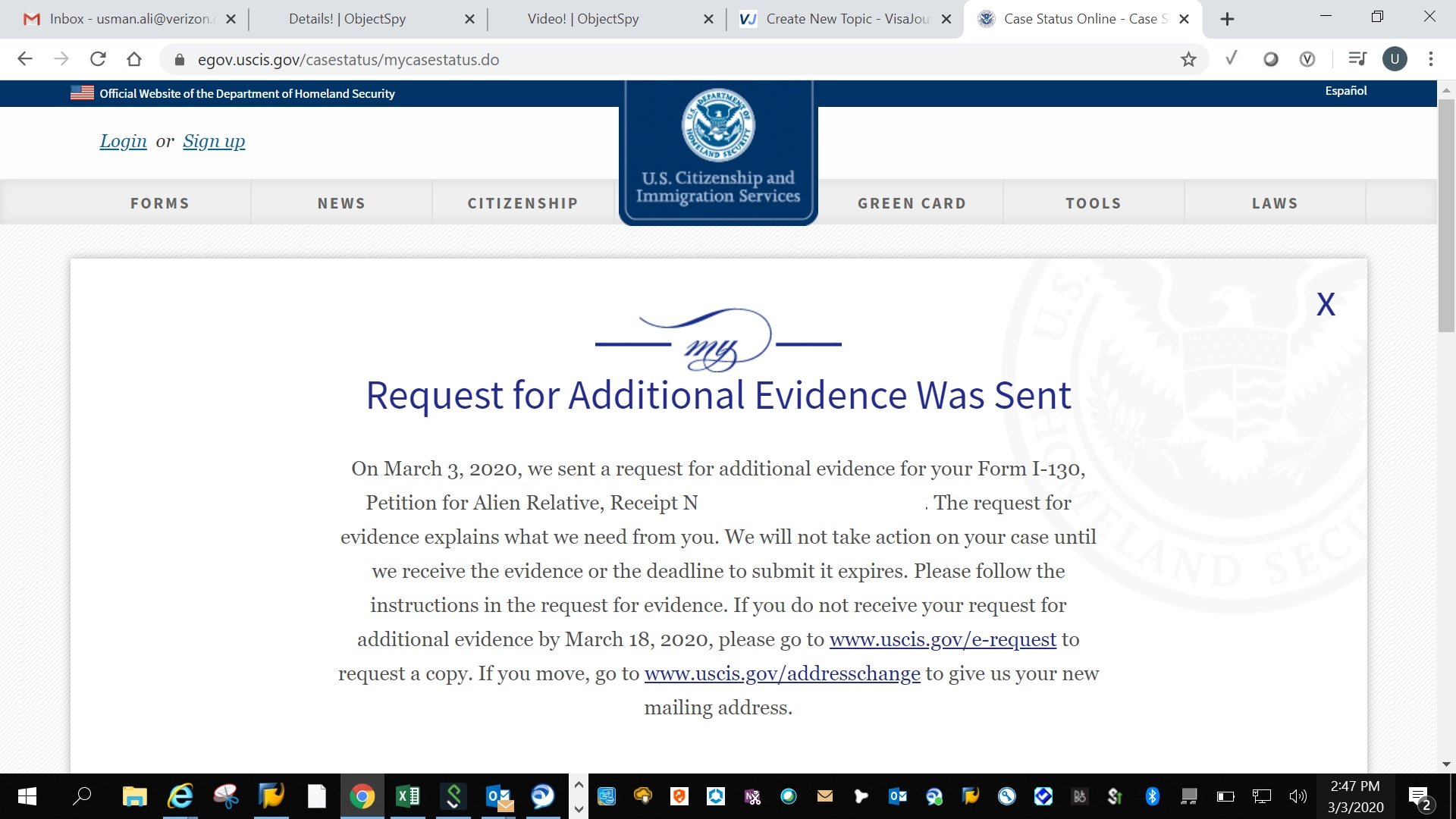**Descriptive Caption:**

This is a detailed screenshot from the official case status page of the Department of Homeland Security's U.S. Citizenship and Immigration Services (USCIS) website, accessible via egov.ucsi.gov. The page features a login and sign-up link located at the top left corner, accompanied by the official blue seal of the U.S. Citizenship and Immigration Services. Below the seal, there are navigational tabs titled 'Forms', 'New Citizenship', 'Green Card Tools', and 'Laws'. 

The main content of the webpage includes a status update for an immigration case, specifically an I-130 petition for an alien relative. The title of the status update is highlighted in blue text, while the detailed message is in black. According to the update, on March 3, 2020, USCIS sent a request for additional evidence pertaining to the case. The receipt number linked to this case has been obscured for privacy. 

The message further explains that this request outlines the necessary evidence required to proceed and that no further action will be taken until the requested evidence is provided or the submission deadline expires. Applicants are advised to follow the instructions included in the request. Additionally, it is noted that if the applicant does not receive the request by March 18, 2020, they should visit the USCIS website to submit an e-request for a copy. Lastly, the message reminds applicants to update their mailing address at USCIS.gov in case of an address change.